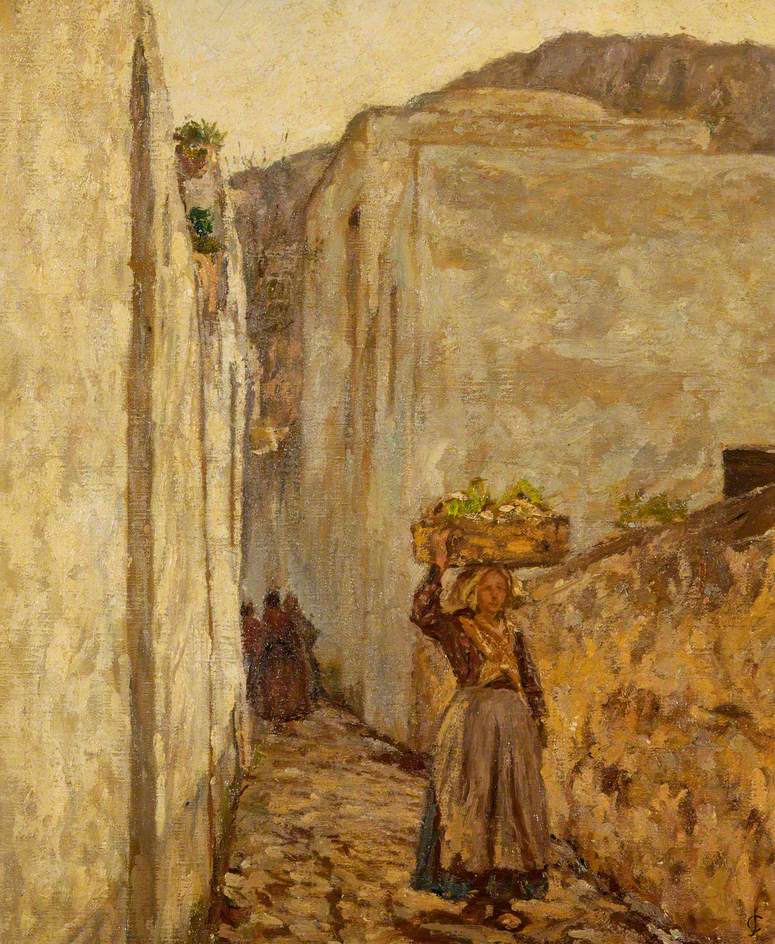In this vibrant painting, a woman dressed in traditional attire walks down a narrow, cobblestone alley in a European village. She balances a large, wooden box laden with fruits or flowers on her head, secured with her right hand. Her attire is ornate, featuring a red, floral-accented top, a bluish-green long dress that reaches the ground, an apron, and sandals. Her hair, shoulder-length, peeks out from beneath a white headscarf. Flanking her path are tan stone buildings, the left adorned with greenery and potted plants at the top. Further back in the painting, other villagers can be seen gathered. The alleyway is bordered by tall concrete or stone walls, leading to a backdrop of towering, rocky mountains under a sky tinted with yellow and blue hues, creating a harmonious blend of earthy and cool colors.